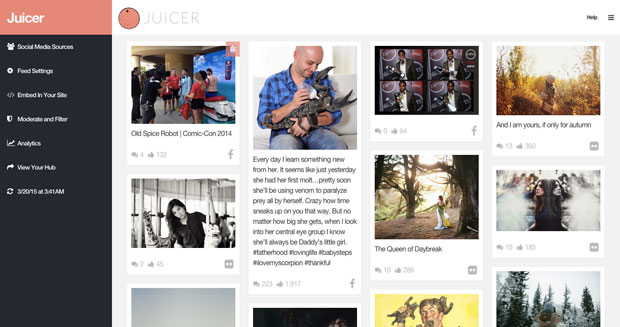This image depicts the homepage of a photo-based website named "Juicer". In the top left corner, "Juicer" is displayed in white text against a pink background. Below, a vertical menu lists various categories: "Social Media Sources," "Food Settings," "Embed in Your Site," "Maximize and Filter," "Analytics," "View Your Hub," and the current date and time, noted as March 3, 2015, at 3:41 AM.

Central to the upper section, slightly left-aligned, the "Juicer" name is reiterated accompanied by its logo—a pink circle that likely represents a fruit. On the top right, the "Help" option is situated next to a hamburger menu icon.

The main content area is filled with square photo thumbnails. In the central square, there is an image of a fair-skinned man wearing a blue checkered shirt and blue pants, holding an animal. To the left of this picture, a group of people are seen actively taking photographs.